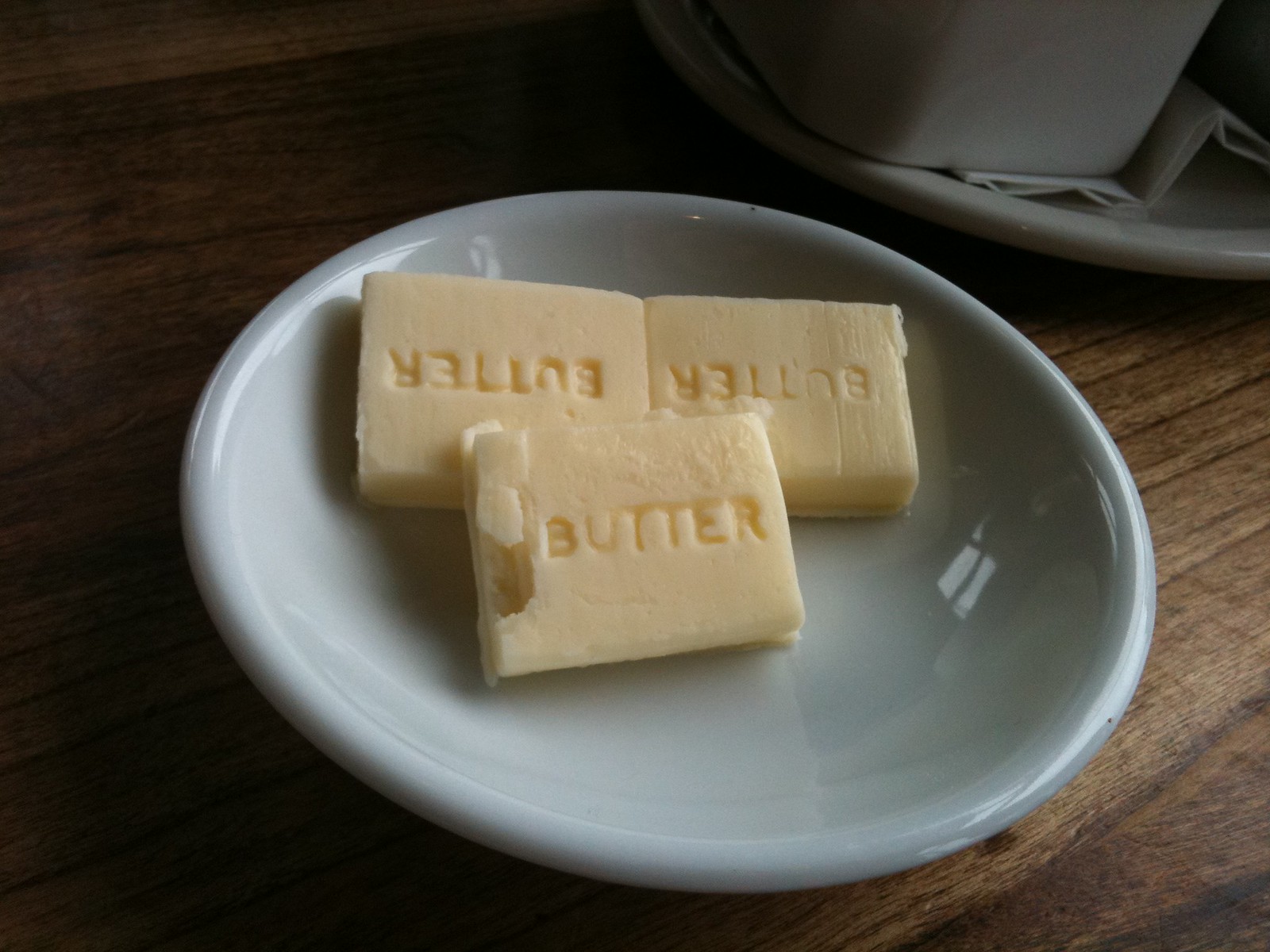The photograph features three rectangular pats of butter on a small, shiny white saucer, which is set on a dark, glossy wooden table. Each piece of butter has the word "BUTTER" embossed in capital letters across the center. The pat in the foreground displays the word correctly, while the two in the background show the embossing upside down. The middle piece has a small chunk taken out of its left side. In the background, partially visible, is another white plate with a white napkin and an indeterminate white container. Shadows cast on the saucer suggest nearby light sources, possibly from a door or window.